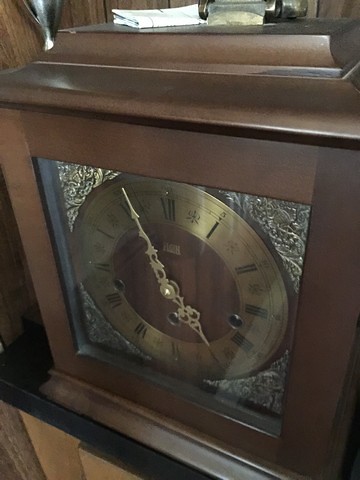This detailed photograph captures the interior of a home or building, featuring a distinctive clock displayed on a wooden platform or end table. The clock itself stands out with its unique structure: a large, square, wooden base painted in a dark, brassy metallic color, reminiscent of a coffin with a lid on top. The clock face is protected by a piece of glass and framed within a circle, creating four embossed triangles at each corner - upper left, upper right, lower left, and lower right.

The round clock face, embellished in brass, is marked with bold Roman numerals in black. The clock hands are highly decorative, fashioned in intricate wire and swirl designs, culminating in a triangular point at the tips. Notably, the hands of the clock, which are golden in hue, are positioned to show the time at approximately 4:56. The wooden frame of the clock has a slight gloss and adds to the overall elegant aesthetic of the piece.